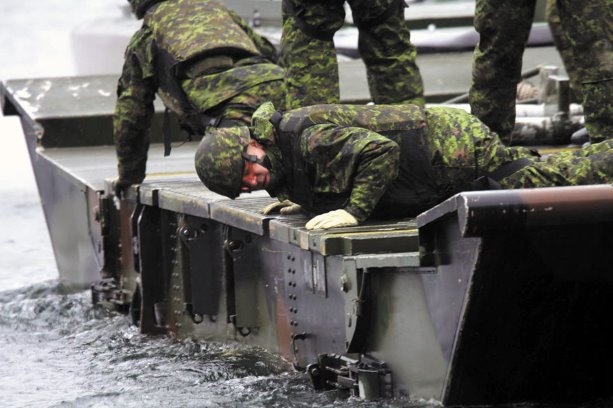The photograph captures a dynamic scene of military men aboard a dark green, possibly black, metal boat navigating through the ocean. The soldiers, dressed in green camouflage gear, helmets, life vests, and white gloves, blend seamlessly into the vessel. The focal point is a soldier laying down on the boat, peering over the edge with his hands palm down, possibly inspecting the water or the boat's machinery. Beside him, another soldier is down on one knee. In the background, the legs of two more standing soldiers are visible, indicating their alert presence as the boat moves through the waves.